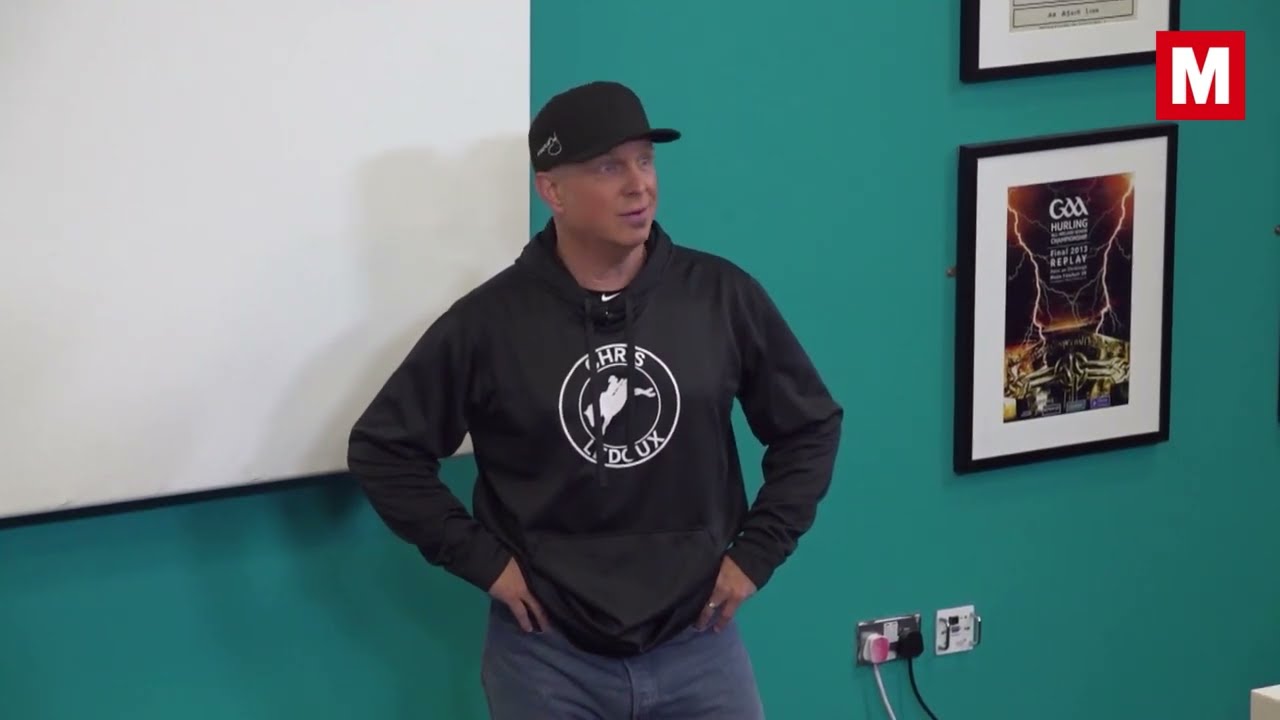The image captures a middle-aged man with white skin and a tan, standing confidently against a light teal green wall, framed by a multitude of details that paint a vivid scene. He has no visible hair under his black baseball cap and is clean-shaven. Dressed casually yet purposefully, he sports a black hoodie adorned with a white circular logo featuring the name "Chris LeDoux" and an emblem resembling a silhouette of someone riding a horse or bull. Accompanying his hoodie are a pair of jeans. With his hands placed firmly on his hips, he appears to be engaging in a lecture or presentation. 

To his right, between him and a couple of framed pictures with black frames, are electrical outlets with various items plugged into them, suggesting a higher caliber not typically found in a home setting. Behind his right shoulder is the visible corner of a large white presentation screen, while the upper right corner of the image features a small red box with a prominent white letter "M". The overall ambiance of the setting, combined with his attire and stance, suggests a moment of shared knowledge or instruction, with the man as the focal point around which these meticulously noted details revolve.